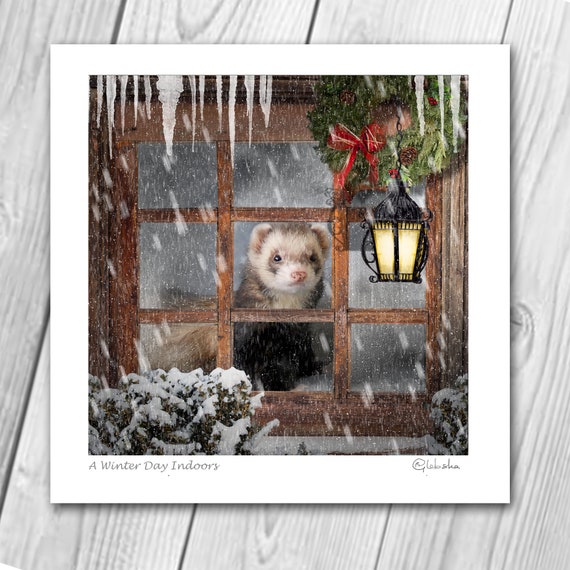This photograph presents a highly realistic art print or digital rendering on cardstock, placed on a tabletop with a striking white and gray wood grain pattern. The main image occupies most of the card, depicting an exterior house scene during wintertime. Dominating the scene is a window with a wooden frame divided into nine panes. Beneath the window, snow-laden shrubs add to the wintry ambiance, with falling snow creating a sense of cold serenity. Icicles hang from the roof edge at the top of the window, emphasizing the frigid weather. On the upper right corner of the window, a Christmas wreath and an accompanying lantern are visible, contributing to the festive feel. Intriguingly, looking out from the middle pane is a small ferret, adding a charming focal point to the winter scene.